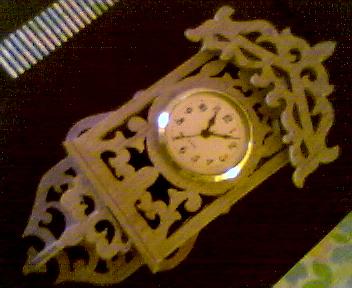This color photograph depicts an elaborately ornate antique clock set at around 11:08. The clock appears to be tilted approximately 45 degrees to the right. The clock face is white, featuring traditional numbers 1 through 12, encased in a gold-colored frame with intricate scrollwork at the top and around the sides, culminating in a rectangular wooden housing that suggests an almost Indian style. The clock's structure includes a hooded top, resembling the roof of a house, yet lacking an opening for a cuckoo as found in traditional cuckoo clocks. The entire piece rests on a black surface that creates contrast but blends into a predominantly dark backdrop. In the bottom right corner, a faint floral patterned wallpaper hints at an environment, while white-striped areas near the top left add texture to the scene. The photograph is of low resolution, making it somewhat grainy and blurry, which adds to its vintage aesthetic.